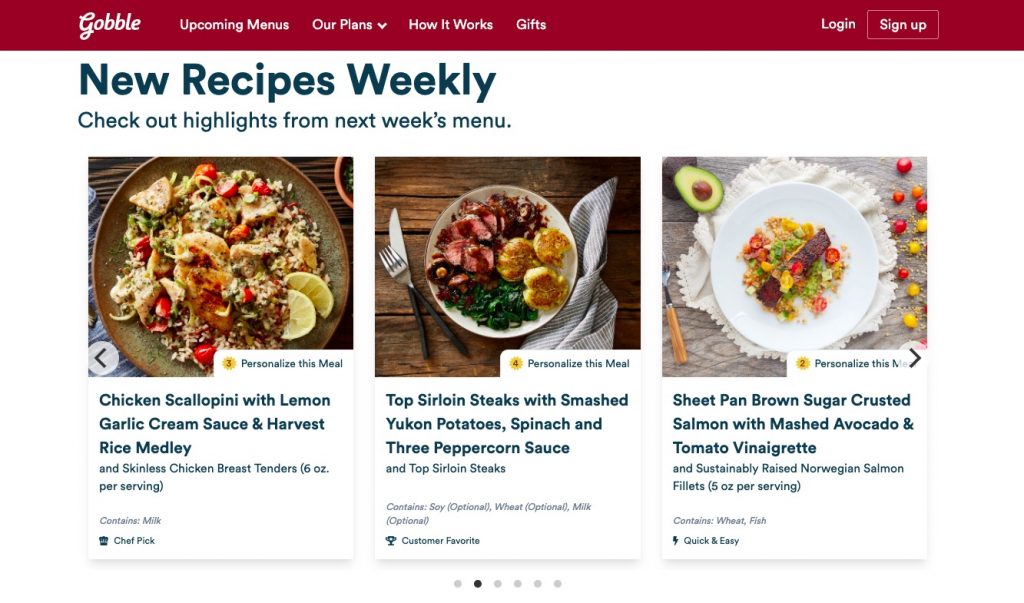The webpage in the image appears to be from "Gobble," a food or meal delivery service. The top of the webpage features a horizontal dark red banner. On the left side of the banner, "Gobble" is displayed in white lettering. To the right of "Gobble," also in white, are options for "Upcoming Menus or Plans" with a downward-pointing arrow, "How It Works," "Gifts," and on the far right, "Log In" and "Sign Up."

Below the banner, against a white background, a message in dark letters reads: "New Recipes Weekly, Check Out Highlights from Next Week's Menu." This section features three images of different plated meals.

1. The first image on the left showcases "Chicken Scallopini with Lemon Garlic Cream Sauce and Harvest Rice Medley." The description notes it includes "Skinless Chicken Breast Tenders, six ounces per serving," and mentions that it contains milk. This dish is also labeled as a "Chef Pick."

2. The middle image depicts "Top Sirloin Steaks with Smashed Yukon Potatoes, Spinach, and Three Peppercorn Sauce." The ingredients listed are "Top Sirloin Steaks," with an emphasis on optional allergens: "Contains Soy Optional, Wheat Optional, Milk Optional." The image shows a plate of food with a fork and a knife placed on the right.

3. The third image on the right displays "Sheet Pan Brown Sugar Crusted Salmon with Mashed Avocado and Tomato Vinaigrette." The dish includes "Sustainably Raised Norwegian Salmon Filet, five ounces per serving" and notes it "Contains Wheat and Fish." The photograph features a white plate with the meal and half an avocado.